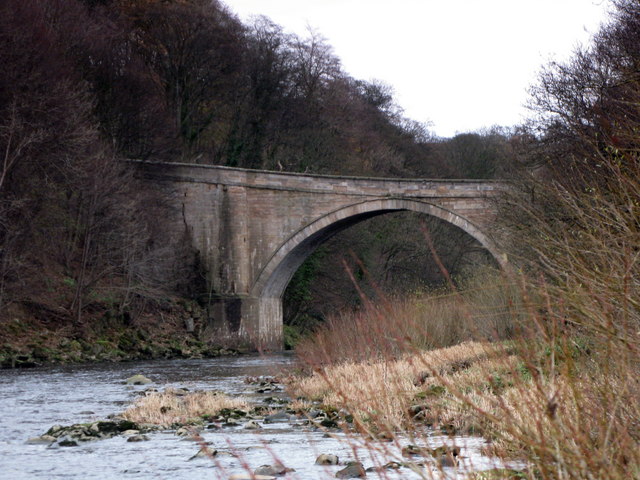The image depicts a rustic footbridge, likely made of stone or brick, stretching horizontally over a shallow stream in a rural area. The setting abounds with natural elements, with overgrown woods and dead branches scattered in the foreground. The water, littered with rocks and weeds, appears tranquil yet shallow, bordered by silty banks. Dead trees are visible to the left of the bridge, creating a dark, muted backdrop that contrasts with the lighter hues of the foliage and the dead weeds emerging from the water. The bridge, positioned centrally in the image, cuts between the serene stream below and the overcast, gray sky above, giving a bleak yet naturistic atmosphere. No text is present in the photo, and the dominant colors are earthy tones of brown, gray, and green, enhancing the somber, tranquil mood of the scene. The perspective suggests the viewer might be standing within the stream, looking up towards the bridge framed by the trees.